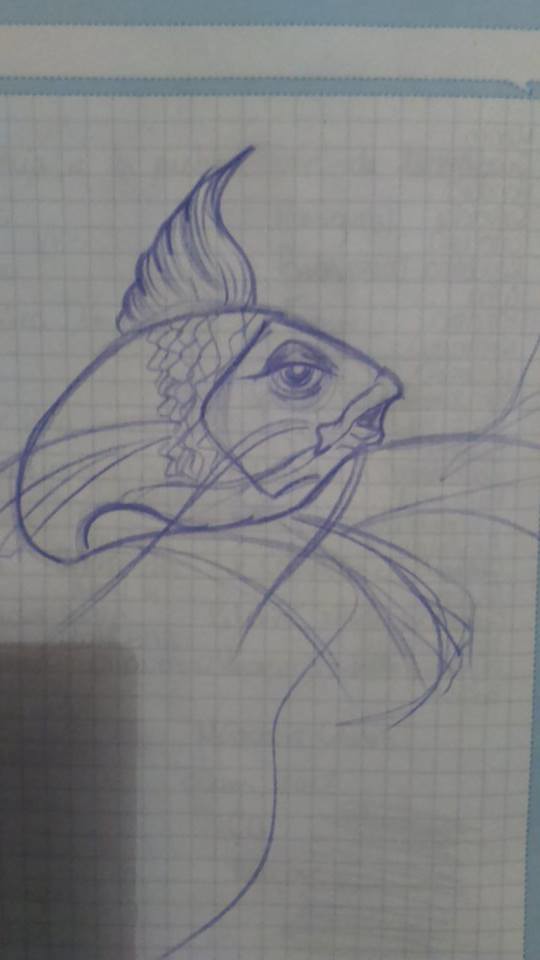This detailed image showcases an ink drawing of a fish, rendered meticulously in blue ink on graph paper. At first glance, the fish, potentially a catfish due to its prominent whiskers flanking its mouth, draws attention. Its eye is lifelike, with half-covered, heavy dark eyelids giving it a somewhat expressive appearance. The lips are outlined, giving the mouth a noticeable definition, and its body is turned, revealing some scales and additional whiskers.

The dorsal fin is distinctively wavy and shaded in with blue, evoking motion as if the fish is swimming. The fin and the other parts of the fish are carefully detailed, though the side fins remain roughly outlined. The fish's abdomen shows swirling lines, possibly an artistic representation of water.

The drawing resides on graph paper, identifiable by its grid of small squares. Of note is the visible blue border on the lower left and top edges of the paper. The top edge features a blue line, a blue bar with a white bar beneath it, and then another blue bar; intriguingly, this white bar resembles a speech bubble, with a small point on its lower right side.

Additionally, there is a shadow in the lower left section, rectangle-shaped as if the image were photographed. These details enhance the ink drawing's depth and the artist's intent, making the entire composition both vivid and engaging.